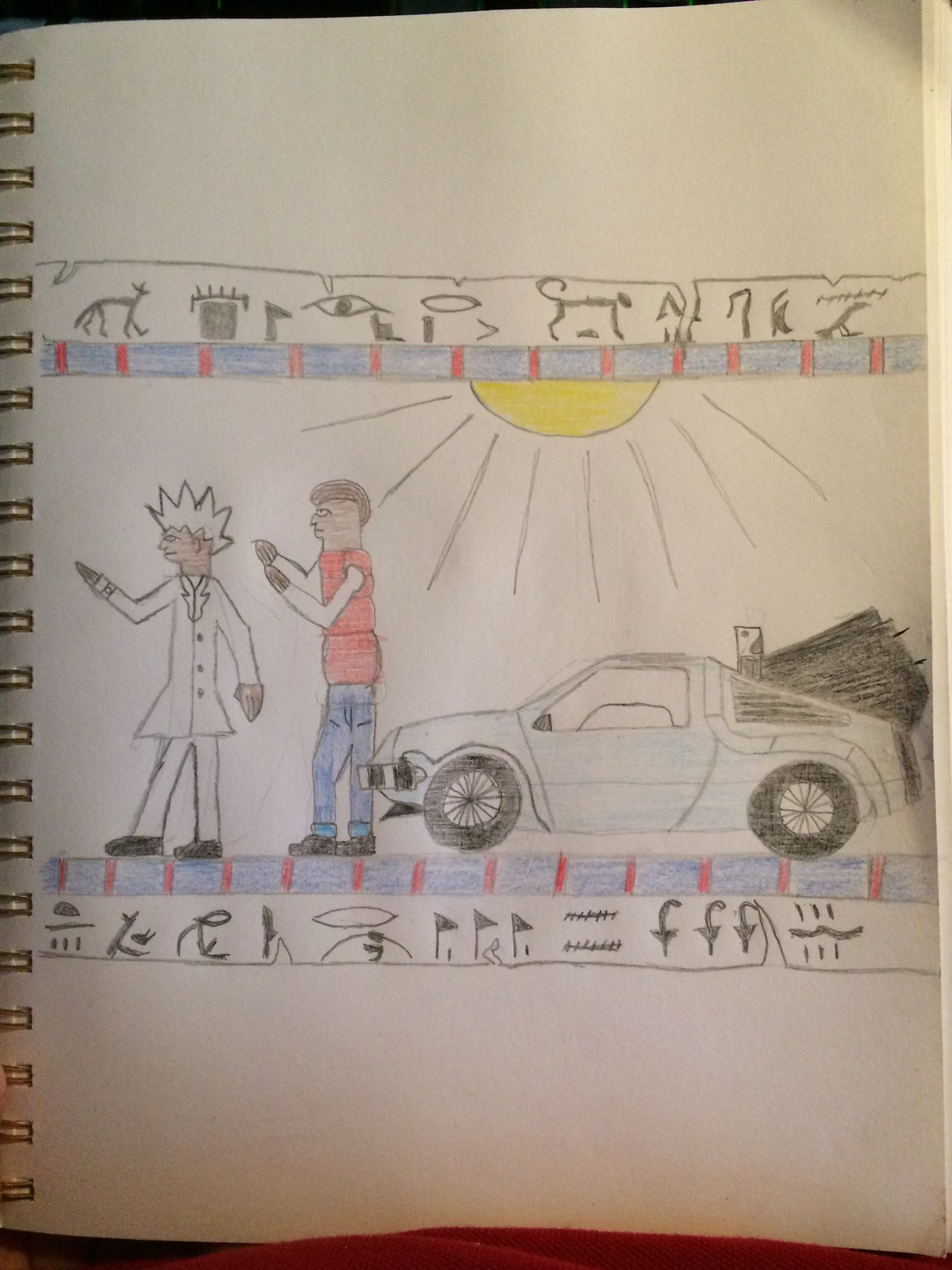This detailed drawing, seemingly from a sketchbook with a spiraled left side, depicts characters from "Back to the Future" in an artistic homage to ancient Egyptian art. 

In the center, rendered with pencils and colored pencils, are two main figures walking towards the left: the character on the left, likely Doc Brown, is adorned with spiky white hair, a white suit with buttons, and black shoes. The figure right behind him, presumably Marty McFly, sports brown hair, a red jacket with white sleeves, blue jeans, and black shoes. A detailed DeLorean car, associated with the "Back to the Future" series, follows close behind them.

The road beneath their feet is blue with red lines. Surrounding the central figures and vehicle are intricate Egyptian hieroglyphics and symbols, including the eye of Horus and various animals, positioned both above and below the central scene. These elements frame a bright sun with radiating rays shining down on the car and characters, enhancing the ancient yet modern fusion of the artwork. Doc and Marty are depicted in a stylized, side-profile manner characteristic of Egyptian art, adding a unique historical touch to this creative illustration.